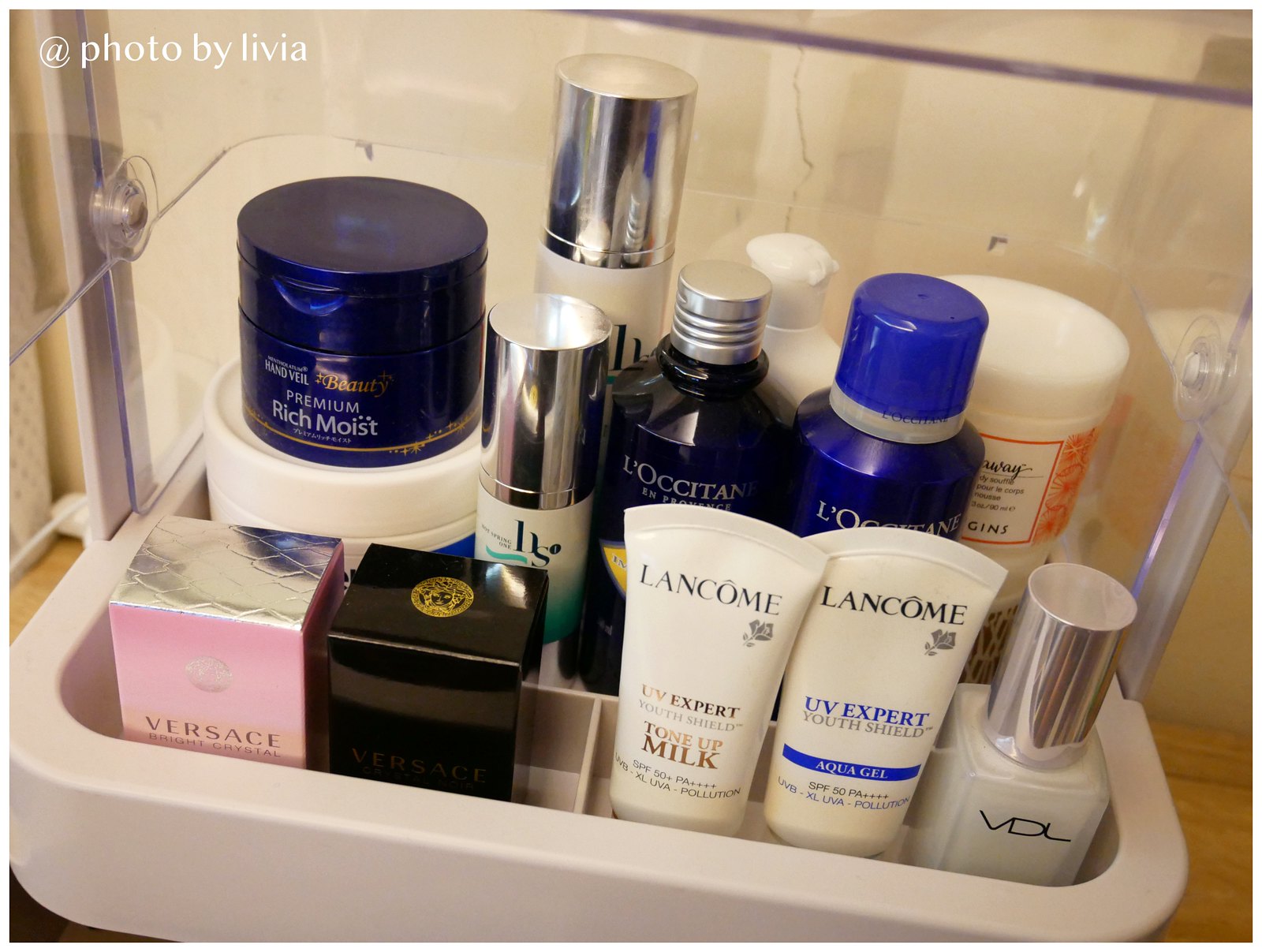The photograph captures a clear plastic storage box brimming with various beauty products. Prominently visible are two tubes of Lancome UV Expert sunscreen. Nestled beside them are two boxed items, one of which is identifiable as a Versace perfume. A bottle of white nail polish stands out amongst the collection. In the background, a diverse array of products is discernible, including two jars, several pump bottles, a variety of other bottles, squeeze bottles, and additional jars towards the right side. The storage box, appearing to have a lid that likely cannot close due to the height of some items, is arranged on a wooden surface with an off-white, possibly eggshell-colored wall in the background. One of the jars is labeled "Premium Rich Moist," though the complete name isn't fully legible. Additionally, there are two bottles from L'Occitane, although their specific contents are unclear.